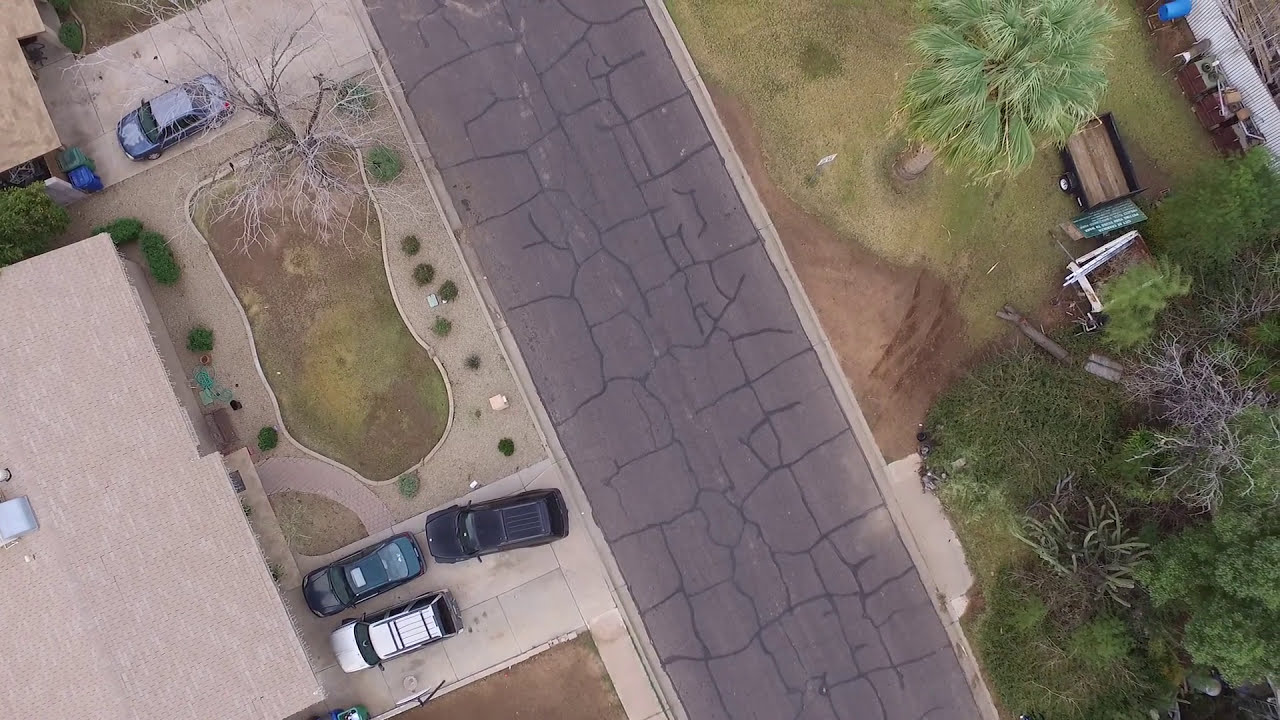In this detailed aerial photograph taken from a drone, we see a cracked asphalt road running diagonally from the top left to the bottom right of the image. The road is heavily lined with cracks, indicating its aged condition. On the left side of the road, a driveway belonging to a house is visible, occupied by three vehicles: one white, one black, and one blue. Slightly further down and close to the center of the image, there is another driveway with a bluish-colored vehicle. Between these two driveways lies a lawn area covered predominantly with white gravel, interspersed with a few bushes and an irregularly shaped patch of dirt and grass that features a large leafless tree at its center. 

On the left side of the image, the rooftops of a couple of buildings are partially visible, while on the right side, in the top right-hand corner, there is a fence cluttered with various items, giving an impression of accumulated junk. Also visible within this more cluttered yard area is an empty wagon and a green and white sign. The image, captured on an overcast day without any noticeable shadows, presents a clear, detailed view of this residential neighborhood, marked by aged infrastructure and a mix of nature and human elements.